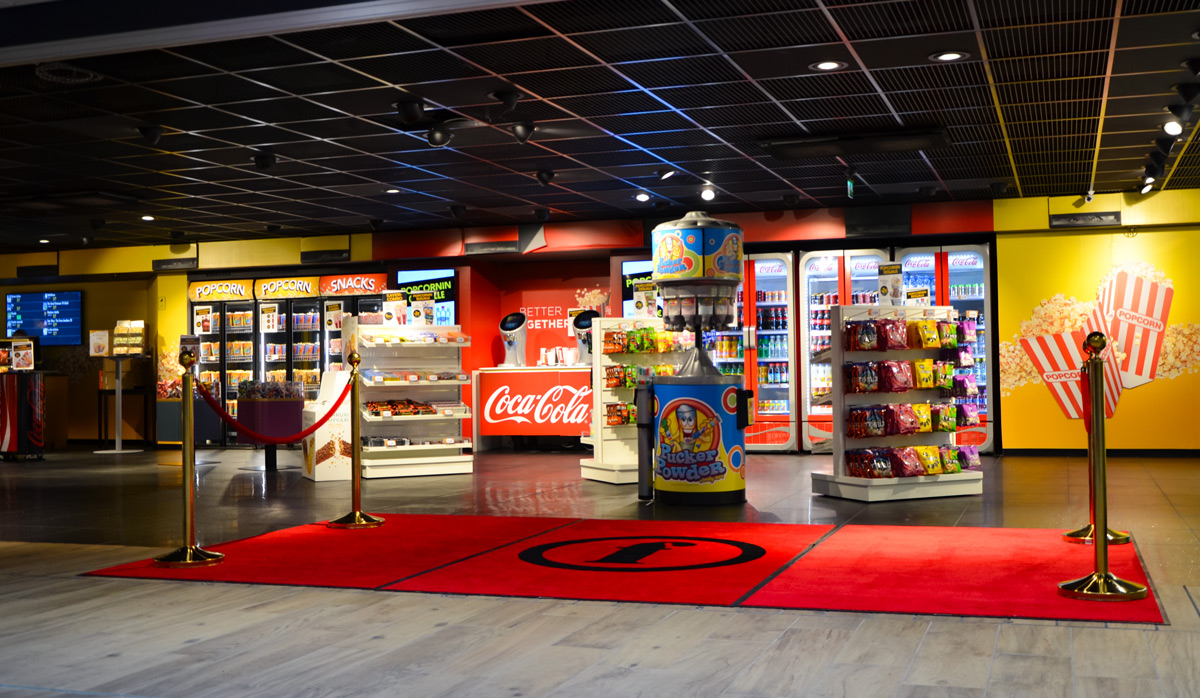The image captures the vibrant lobby of a high-end movie theater, designed for both aesthetics and functionality. Dominating the center of the scene is a distinct red carpet embellished with a black circular logo featuring a lowercase 'f'. Flanking the carpet are gold crowd control barriers connected by slouching red velvet ropes, guiding patrons towards various snack kiosks.

To the left and right of the red carpet, additional details enrich the overall scene. The foreground showcases a light brown wooden floor transitioning into a sleek black floor, partially defining the space. Various kiosks populate the background: on the left, there's a black screen with blue text, and a gray table exhibiting white and yellow items. Closer to the center, another kiosk branded as 'Pucker Powder' displays colorful polka dots and offers sour candy; a whimsical man in a tin hat adorns its top.

On the far left, several black refrigerators stocked with an assortment of sodas stand against a backdrop featuring the iconic red Coca-Cola logo. A gray table with unidentified items and a Coca-Cola drink creation area suggest multiple beverage options. Towards the left, there is also a dedicated area for snacks and popcorn, with signage in red and white stripes, clearly labeled "popcorn" in red on a yellow background.

In the middle to the background, you can spot more candy stands with organized racks filled with brightly wrapped candies in hues of yellow, red, blue, and green. In the far background, several coolers labeled "snacks" and "popcorn" contain additional refreshment options, continuing the theme of indulgence.

Above it all, the ceiling features a combination of black squares and silver steel grids, contributing to the modern, upscale ambiance of the movie theater lobby. The absence of people suggests either an off-peak time or a fully automated service area, elevating the sleek and sophisticated environment.